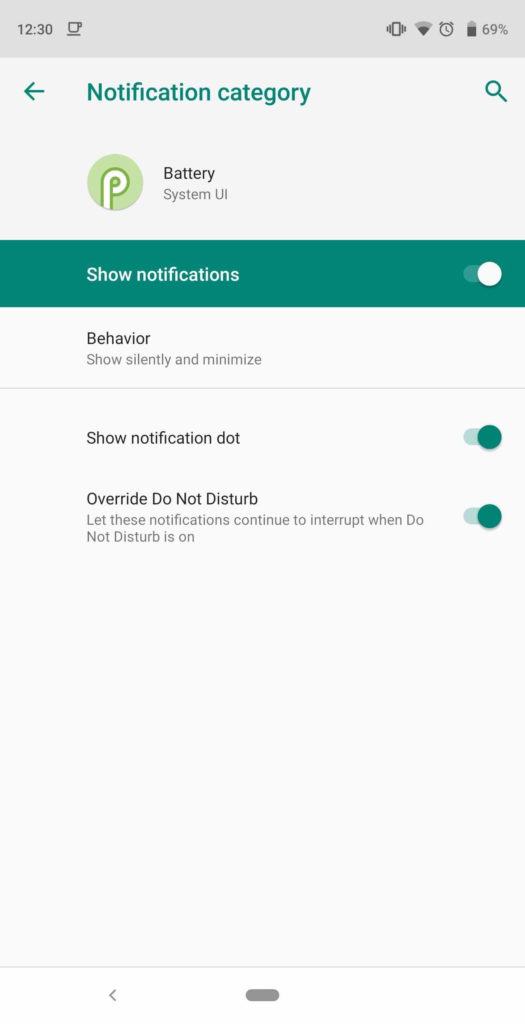In the image, a notification from a smartphone is displayed. The top portion features text reading "Notification category" in a green font, flanked by a back icon on the left and a magnification glass (search icon) on the right. Below this, another text reads "Battery, System UI," accompanied by an icon to its left—a light green circle with a white "P" outlined in green inside it.

Further down, white text reads "Show notification," with a matching white toggle switch to the right, which is turned on. "Show notification" is also set against a green background. Below that, the text "Behavior, Show silently and minimize" is noted.

Near the bottom of the image, another option is displayed: "Show notification dot," with an enabled toggle switch to its right, rendered in green. The final piece of text says "Override Do Not Disturb: Let this notification continue to interrupt when Do Not Disturb is on," accompanied by another green, active toggle switch on the right.